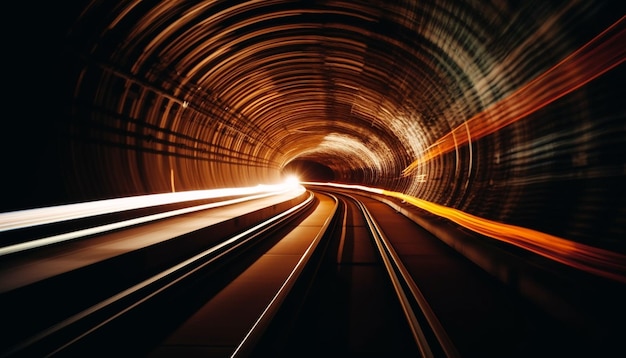This hyper-realistic digital creation, resembling an AI-generated image or heavily photoshopped photograph, captures a dramatic scene inside a wide-stretched oval train tunnel. The perspective places the viewer down on the dark, shadowy tracks in the foreground, which transition into burnt orange and darker brown as they recede into the distance. The tunnel, lined with indentations around its roof's circumference, showcases an evocative time-lapse effect created by streaks of light. On the left, a bright white line ends in a bulb-like flash, suggesting the headlights of an oncoming train illuminated with hints of yellow. On the right, the lights transition from orange to yellow to white, possibly representing taillights of a departing train. These vibrant streaks curve towards the left at the tunnel's end, where a radiating bright light signifies an approaching or receding train. The overall illumination reveals the service walkway on either side of the track, characterized by coppery hues, silver, and sepia tones, enhancing the surreal, action-packed atmosphere of the scene.